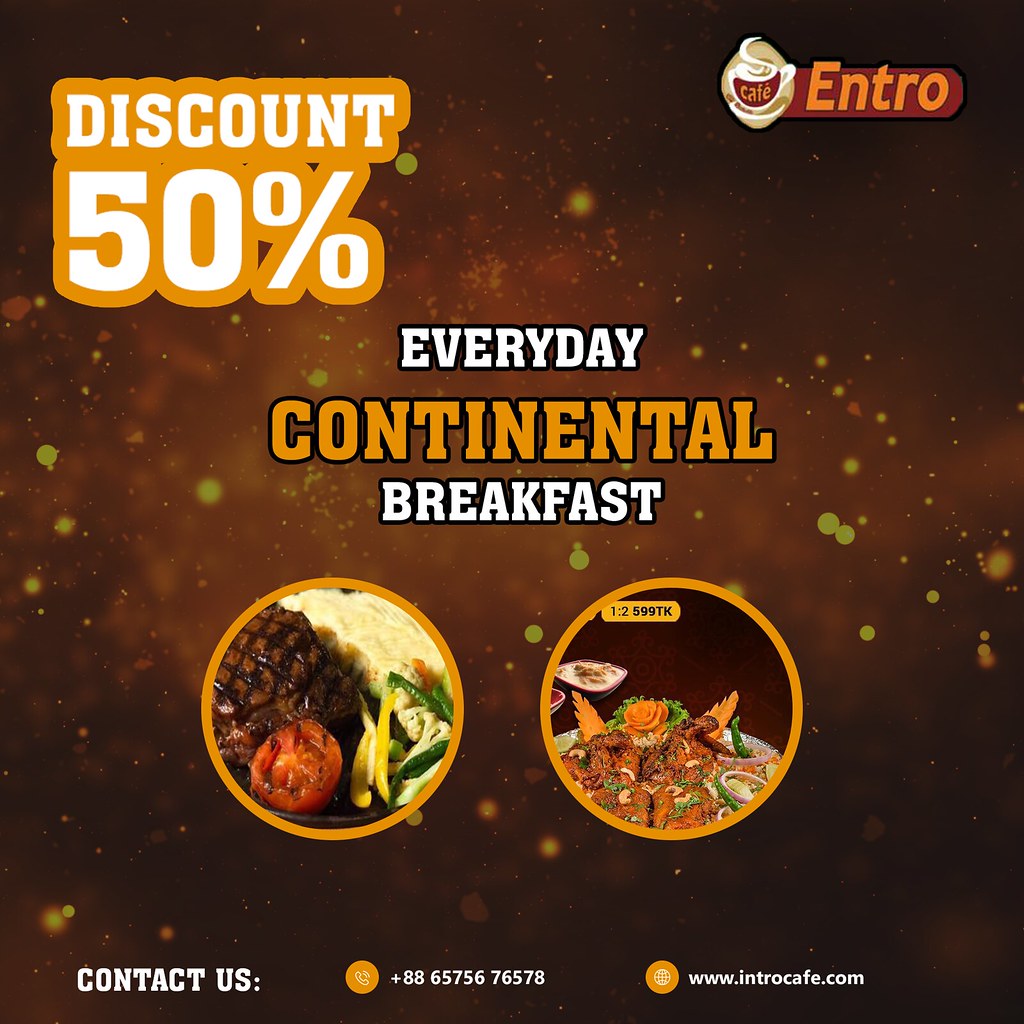The flyer is an advertisement for Entro Cafe, featuring a dark brown background with a textured, bubbly appearance and yellow bubbles spread throughout. In the top right corner, a graphic of a steaming coffee cup labeled "CAFE" is placed alongside the word "ENTRO." The top left corner prominently displays "DISCOUNT 50%" in bold white letters against an orange background.

At the center of the flyer, the text reads "EVERYDAY CONTINENTAL BREAKFAST," with "Everyday" and "Breakfast" in white letters and "Continental" in a yellowish-gold hue. Below this text, there are two circular images of food: the left image features a steak accompanied by a grilled tomato, mashed potatoes, and vegetables, while the right image is less clear but still depicts food.

The bottom section of the flyer states "CONTACT US" in white letters, with icons of a phone and a web next to respective contact details. The phone number provided is +886-5756-76578, and the website is www.entrocafe.com. The flyer also features scattered light spots in the background, adding a sparkling effect.